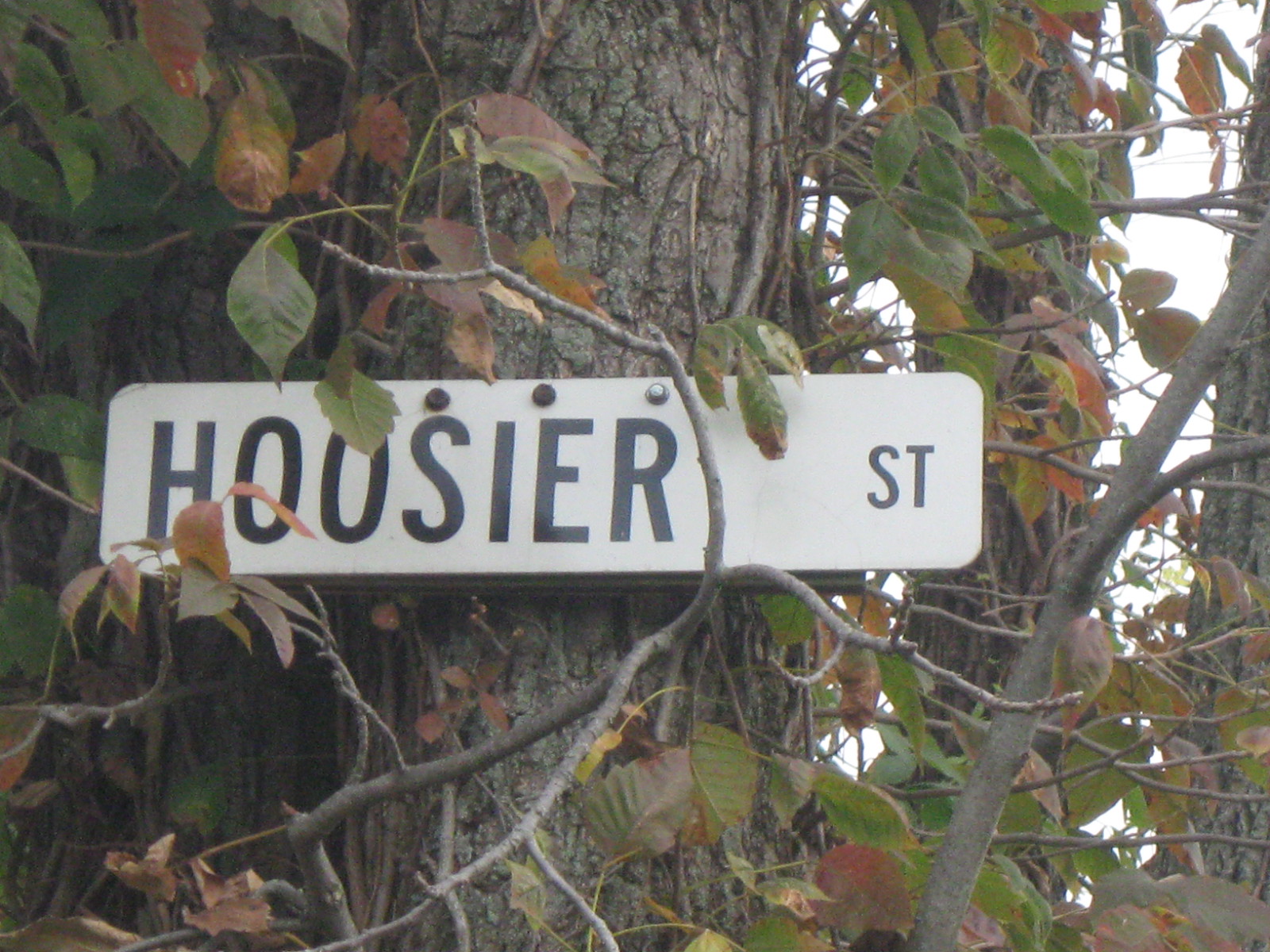This is a close-up photograph taken outdoors, capturing a street sign affixed to a tree. The sign reads "Hoosier Street" in uppercase black lettering on a long, narrow, white background. It is attached with three screws, two of which appear old and rusty, while the third one looks newer and silver. The tree, about a foot wide in diameter, has dark brown bark with textured patterns. Surrounding the tree are branches with leaves that are mostly green, but some are beginning to turn orange-brown, indicating early fall. Sunlight filters through the foliage, adding a natural brightness to the scene. The leaves are abundant and envelop parts of the tree, suggesting the passage of seasons.